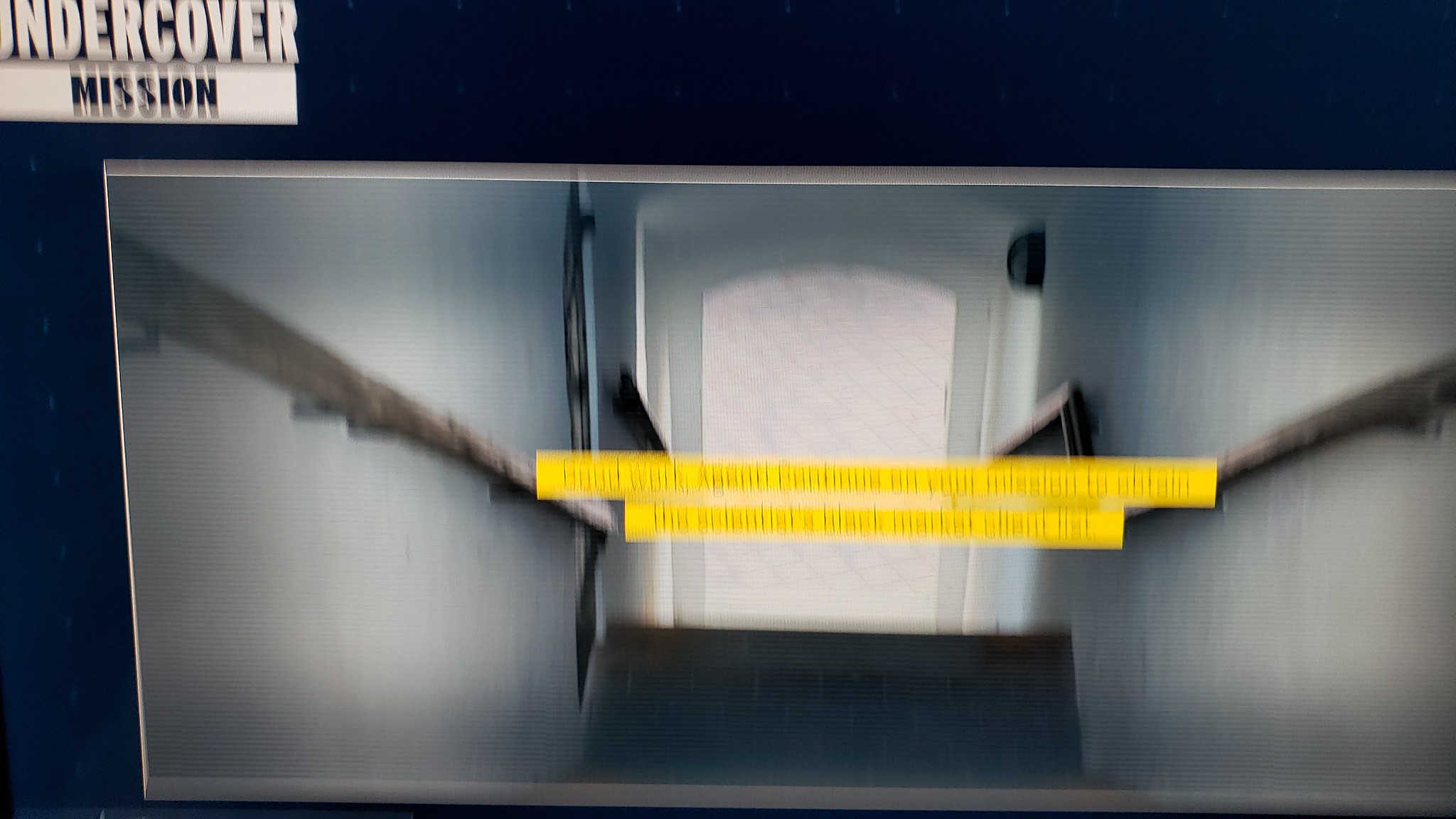In this image, a stairwell is captured from a low vantage point, looking upwards towards another level. The focal point is a central rectangular window adorned with an arched top, which allows an abundance of bright, white light to flood into the space. Flanking the white walls on both sides of the stairs are sleek handrails that first run parallel to the platform before dropping down to follow the line of the steps, guiding the viewer's eye upwards. At the upper landing near the illuminated window, the hallway extends in both directions, suggesting a larger architectural space beyond.